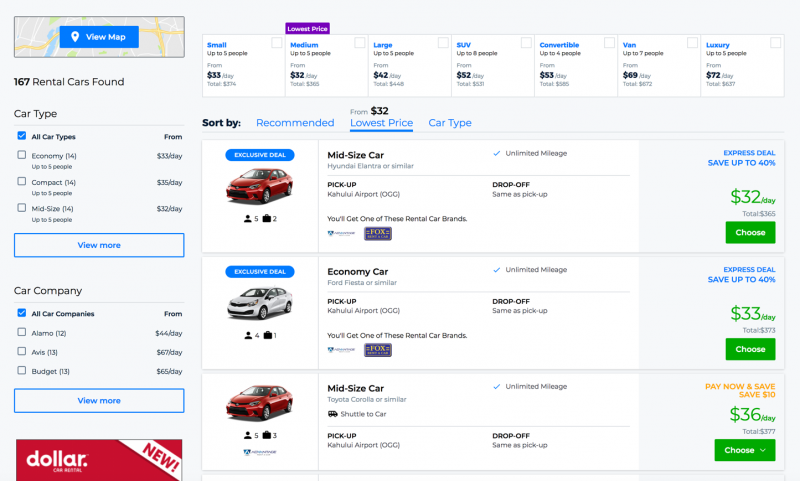The image showcases a rectangular interface with a background in light gray, extending horizontally from left to right. On the left side, there's a prominent column titled "View Map" that includes a background map graphic. Below this map, the column states "167 rental cars found," followed by a series of filter categories. 

The first filter, labeled "Car Type," indicates that all car types are selected, with additional options for economy, compact, and midsize, along with a link to view more options. The next filter, "Car Company," shows that all car companies are selected, and lists Alamo, Avis, and Budget, again with an option to view more choices.

At the bottom of the column, a red advertisement features white text reading "Dollar."

To the right of the filters, the main section of the interface presents various car rental choices. At the top, there is a category for selecting car sizes based on the number of passengers. Options include up to 5 people, 8 people, up to 4 people, up to 7 people, and descriptions such as luxury, van, convertible, SUV, large, medium, and small. The medium-sized option is noted as having the lowest price per day.

Three specific car listings are displayed, each with detailed information. On the far right of these listings, the prices are highlighted, with the "Lowest Price" category currently emphasized.